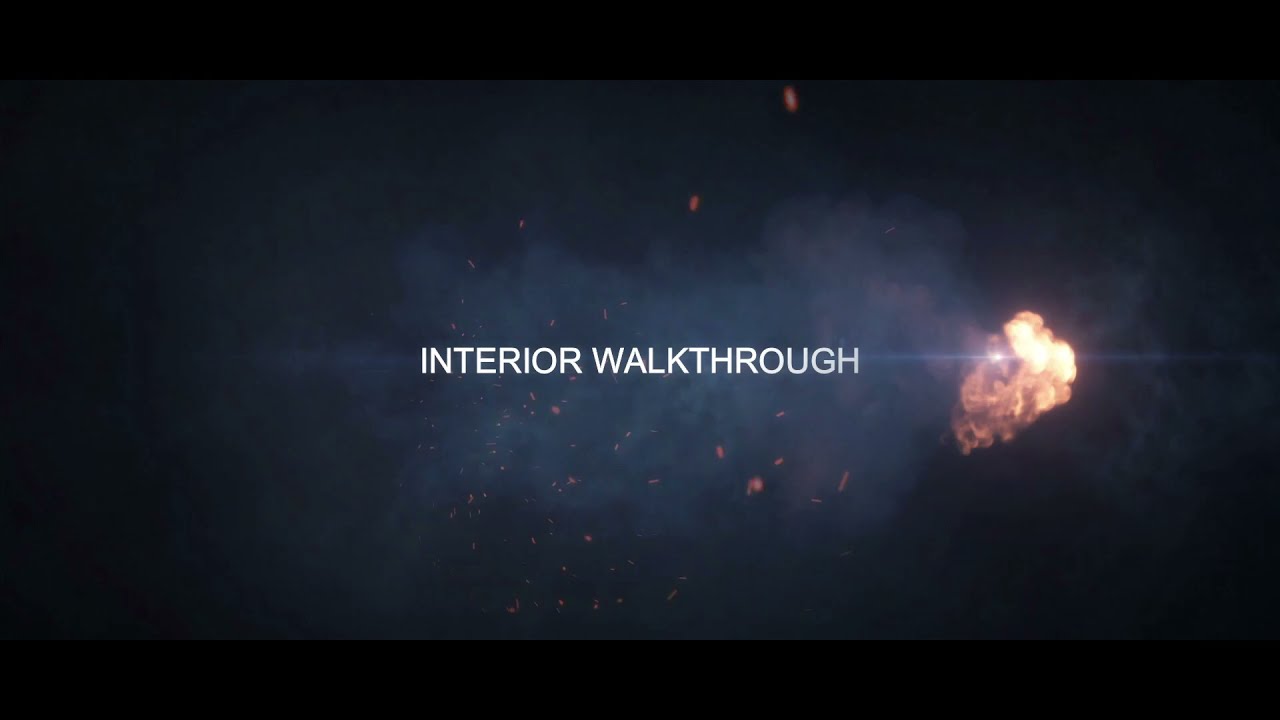This image is a detailed and dramatic digital photograph, resembling a space-themed poster, with a wide rectangular format featuring black bars at the top and bottom. In the center of the image, against a backdrop that mimics a deep space scene, are white, all-capital letters in a sans-serif font, likely Arial, spelling out "INTERIOR WALKTHROUGH." The backdrop includes a hazy cloud, and to the right, there's a small, rocky asteroid with sunlight glinting off its surface. The scene includes red-tinted nebulae and scattered white dots evoking distant stars or galaxies. Center-right, the image depicts a striking explosion with bright orange and yellow flames and accompanying smoke, creating a dramatic fiery burst that contrasts against the dark space. Little embers of fire can be seen above and below the central text, adding to the intensity of the explosion and enhancing the otherworldly atmosphere of the scene.